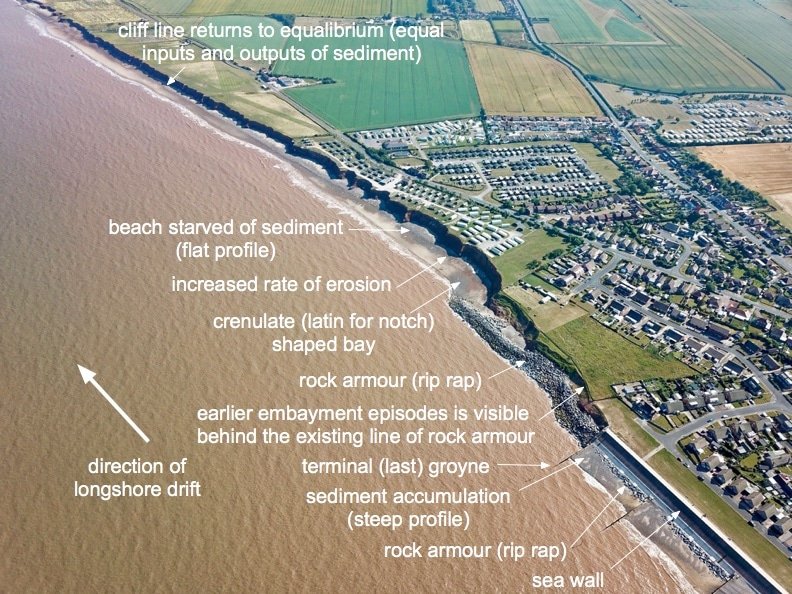This aerial photograph captures a dynamic coastal landscape featuring a shoreline, a suburban city, and an array of fields. The shoreline, demonstrated by brown sand and water, displays various signs of erosion and coastal management efforts. Text annotations with arrows elaborate on these coastal processes: 

- At the upper edge, "Cliffline returns to equilibrium (equal inputs and outputs of sediment)" points to a relatively straight cliffline.
- Below, "Beach starved of sediment (flat profile), increased rate of erosion, crenulate (Latin for notch) shaped bay" highlights areas of significant sediment loss and erosion.
- Further down, "Rock armor (riprap)" indicates strategic placements of rocks aimed at countering erosion.
- Another note reads, "Earlier embayment episodes visible behind the existing line of rock armor," revealing previous coastal changes.
- Additionally, the term "Terminal (last) groyne" and "Sediment accumulation (steep profile), rock armor (riprap)" suggests the construction of structures to trap sediment and stabilize the area, leading to a steeper beach profile.
- At the bottom, "Seawall" depicts another protective measure against coastal erosion.
- Lastly, an arrow pointing left marks the "Direction of longshore drift," indicating the prevalent movement of sediments along the coast.

In the background, there's a visible cityscape lined with houses and streets, typical of suburban development. Further back, several fields vary in color, including dark green, yellow, and mixtures thereof, suggestive of agricultural usage. The top part of the image features a wild green field. This detailed caption underscores the ongoing battle against coastal erosion and the structural attempts to mitigate it, framed by urban and rural land uses.